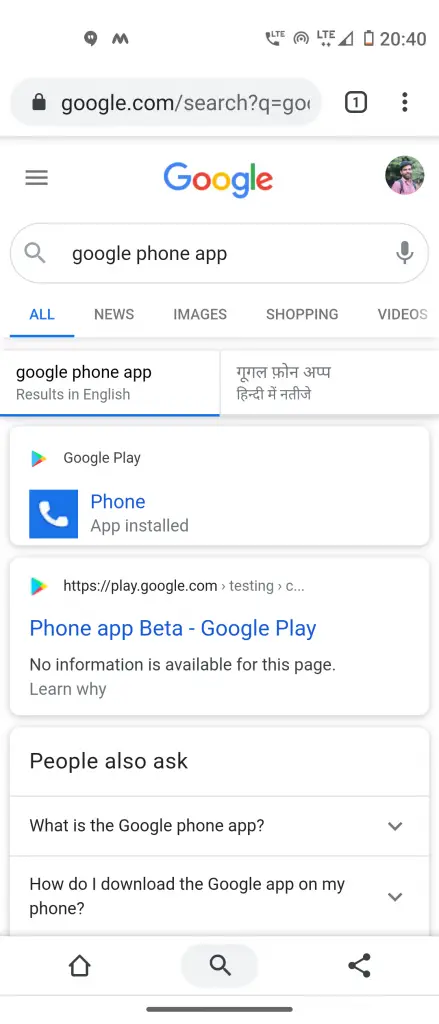A detailed screenshot from a cell phone displays multiple elements of a Google search page. At the top of the screen, various icons are visible including those for Gmail and LTE connectivity, while the battery icon shows a critically low level. The time displayed is 20:40. The search bar at the top reads "google.com/search?q=GO," though the rest is cut off. Beneath the search bar, three horizontal lines, and the word "Google" are visible next to a small circular photograph of a man facing the camera.

Below the Google logo, the active search bar contains the query "Google phone app." The search options available are "All" (which is selected), "News," "Images," "Shopping," and "Videos." The search results are primarily in English, but also include some text in what could potentially be Urdu. The first result indicates the “Google Play phone app is installed” with a URL pointing to "https://play.google.com." It includes a message about a "Phone app beta Google Play" with no additional information available, along with a link to "Learn why."

Further down, the section “People also ask” features questions such as "What is the Google phone app?" and "How do I download the Google app on my phone?" At the bottom of the screen, a navigation bar displays three icons: home, search (which is highlighted), and share.